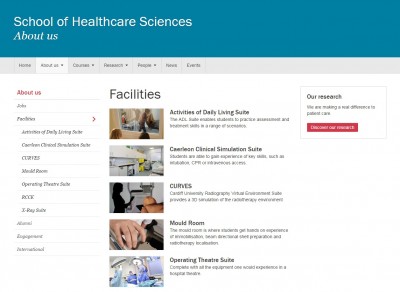The landscape-format, color screenshot captures a cropped view of a website’s "About Us" page for the School of Healthcare Sciences. Positioned in the center of the page is the "Facilities" heading, listing key features such as Activities of Daily Living, Curves, the Mold Room, and the Operating Theater Suite. The site layout reveals seven tabs, with "Home" and "About Us" being discernible, and the latter currently selected. The central content is set against a clean, white background. A distinctive marine blue banner at the top prominently displays the School of Healthcare Sciences title, adding a professional touch to the web page’s design.